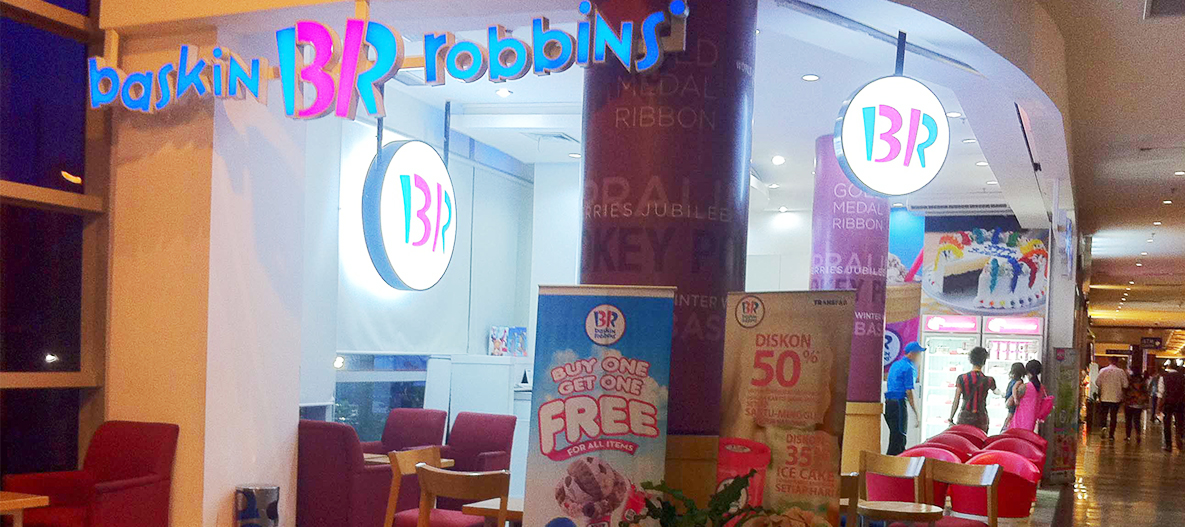This image captures a bustling Baskin Robbins store located inside a shopping mall. The storefront is vibrantly branded with the iconic Baskin Robbins logo, featuring "Baskin" written in light blue, "Robbins" in the same shade, and the distinctive "BR" in a mix of pink and blue. Prominently displayed in the center above the entrance is a white circle bearing the "BR" logo, along with lighted bulbs also showcasing the logo.

Inside the shop, noticeable features include red and brown chairs, one positioned under an uninhabited window. The store is lively, with a male worker dressed in a blue outfit and cap attending to three female customers—one in a pink dress and another in a red dress. There are two prominent promotional signs at the front of the store: one advertising a "Buy One, Get One Free" deal in blue, pink, and white colors, and another offering "50% off" and "35% off" discounts, possibly on ice cream cakes, indicated by accompanying Baskin Robbins logos and images of an ice cream cake adorned with colorful, rainbow-like icing.

The background reveals the broader mall environment, with several people walking past the store and down a hallway, adding to the dynamic scene. This detailed visual effectively merges the shared elements from the different descriptions to provide a comprehensive and vivid depiction of the Baskin Robbins store and its surroundings.